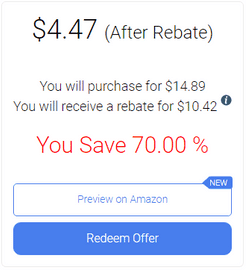In the image, the top section prominently displays a final price of $4.47, enclosed within parentheses, accompanied by the phrase "after rebate." Beneath this, the text details the purchase and rebate process: "You will purchase for $14.89, you will receive a rebate for $10.42." To the right of the $10.42 amount, there is a circular icon with a lowercase 'i' inside, indicating further information. Below this, the text highlights a significant discount, stating "You save 70%" in bold, red font, noticeably larger than the preceding text. Underneath this section, there are two interactive boxes. The first box, labeled "Preview on Amazon," has a white background with blue text and is marked with a 'New' tag in the corner. The second box below it, labeled "Redeem Offer," has a blue background with white text.